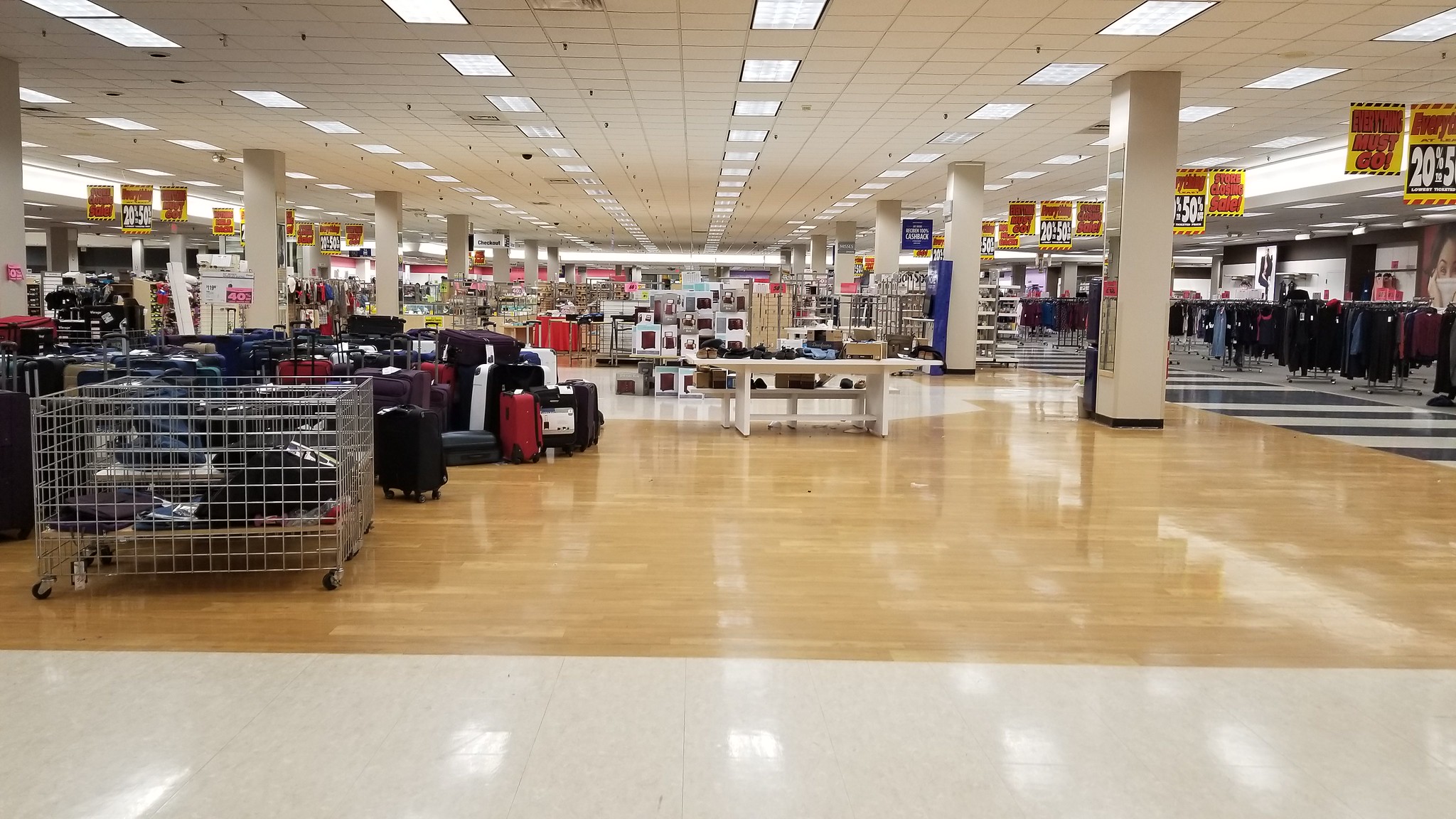This image captures the vast interior of a large department store, likely situated inside a mall. The store features a glossy, light wood floor transitioning to a white surface near the camera, with black and white striped flooring in the distance on the right side. The ceiling is paneled and dotted with square-shaped lights, providing ample illumination throughout the expansive, open space. Tall, light-colored columns are evenly spaced along the store's length, emphasizing its extensive size.

In the background, the store stretches far into the distance, lined with various sections filled with merchandise. The right side of the image showcases numerous circular clothing racks, while the left side displays a variety of suitcases, bags, and potentially some jewelry stands. There is also a cage-like structure holding assorted items on the left.

Prominent red and yellow sale signs are scattered throughout, declaring significant discounts and phrases like "everything must go," suggesting the store may be closing down or having a major clearance sale. Among the merchandise, a sunglasses stand is visible on the right, near one of the columns. The carefully detailed layout and visible signs enhance the impression of a well-organized yet bustling department store, filled with diverse products awaiting eager buyers.